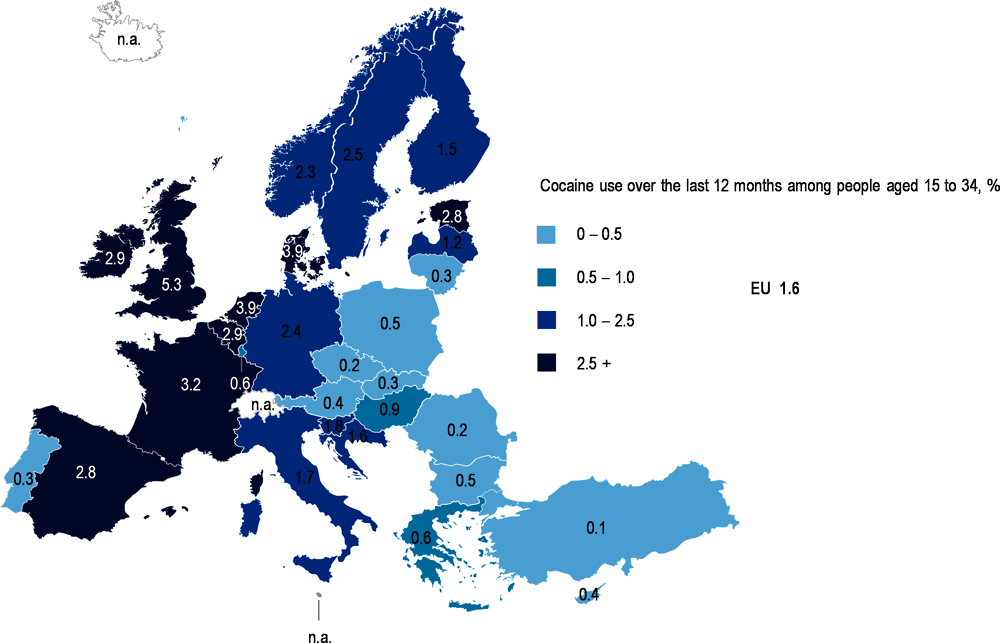This image is a color-coded map illustrating cocaine use over the past 12 months among people aged 15 to 34 across different regions. The map utilizes various shades of blue to represent different percentages of usage. 

- **Light blue** corresponds to regions with 0 to 0.5% reported use.
- **Turquoise blue** indicates 0.5 to 1.0%.
- **Navy blue** represents 1.0 to 2.5%.
- **Dark blue** signifies areas with more than 2.5% usage.

On the right side of the map, there is a legend explaining these color codes. Additionally, it mentions that the average cocaine use within the EU is 1.6%. Each region on the map is shaded accordingly to depict the percentage of cocaine use, providing a clear visual representation of where usage is more prevalent. The rest of the image features a white background that accentuates the color differences on the map.